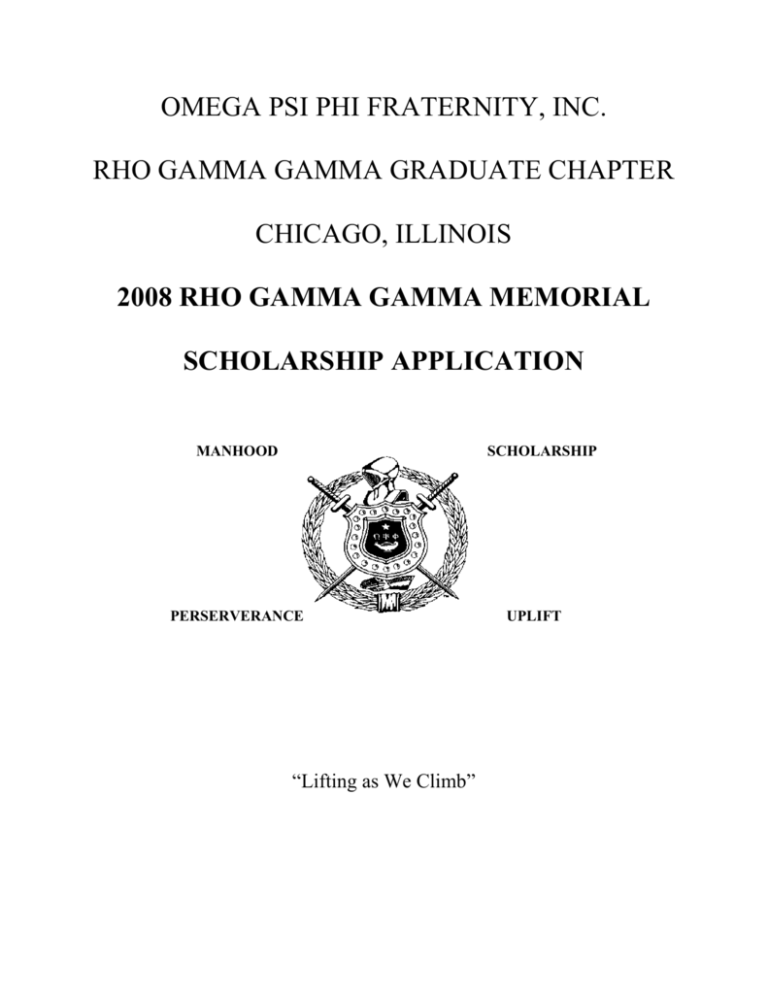The image presents a clean and straightforward design. At the very top center, the text reads "Omega Pi FHI Fraternity, Inc." Beneath this heading is another line of text stating "RHO Gamma Gamma Graduate Chapter." Following this, the location "Chicago, Illinois" is prominently mentioned. Further down, in bold text, the image announces "2008 RHO Gamma Gamma Memorial," immediately followed by "Scholarship Application" also in bold.

A notable feature at the bottom of the image is a detailed logo, presumably representing the associated school or fraternity. This logo depicts a knight facing to the left, equipped with a helmet and armor. In front of the knight, there is a shield. Piercing through the shield are two swords crossed diagonally from the top left to the top right, with only their handles visible at the corners. The shield's edges are adorned with a series of hole-like marks, forming a pattern reminiscent of diamonds. 

Floating around the top and bottom corners of the shield are four significant words: "Manhood" in the top left, "Scholarship" in the top right, "Perseverance" in the bottom left, and "Uplift" in the bottom right, suggesting core values or principles associated with the fraternity or institution.